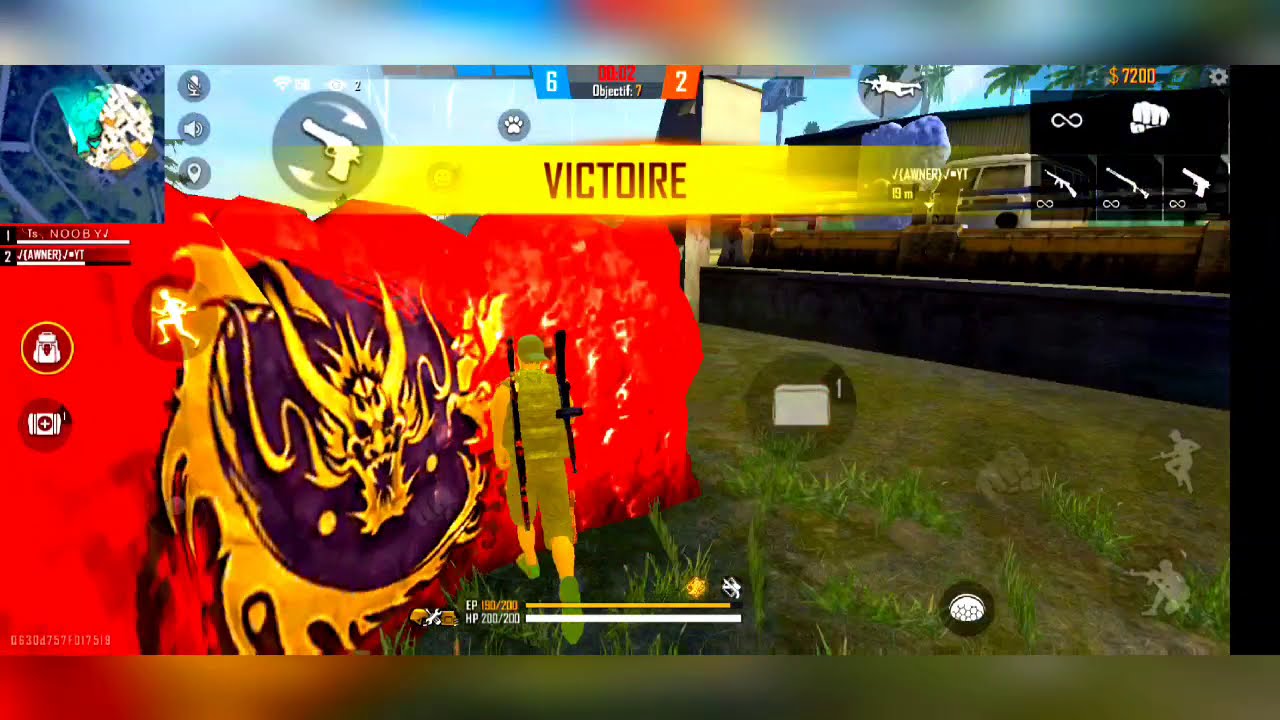The image appears to be a vibrant and dynamic screenshot from a mobile shooting game. Dominating the upper portion of the screen is a prominent "VICTOIRE" banner in a striking yellow color, signaling victory. Surrounding this banner is a variety of game interface elements, including a detailed mini-map in the form of a rectangle with a blue swoosh, which itself is encircled, situated near the top left corner of the screen. Directly adjacent is the image of a gun also encased in a circle, a common control feature for mobile gameplay.

In the lower segment, a dynamic scene unfolds featuring a soldier adorned in a military vest, backwards hat, and shorts. This character is depicted with two long black guns across his back, radiating a glowing yellow hue. He's advancing towards a red flag adorned with a golden dragon head, and a surrounding purple circle with a golden tail, which gives the flag an animated banner-like appearance. This element, combined with the vivid graffiti-like background featuring rich hues of red, yellow, purple, green, blue, and white, contributes to the surreal, collage-like aesthetic of the image.

Also notable in the bottom left corner is an image of a large blue hat with a detailed depiction of a viking character, featuring a yellow swoosh and a vivid red background. Despite the chaotic visual elements, the primary focus is clear: the soldier's action within the game. The blend of interface icons and artistic graffiti work transforms the scene into both a functional game display and an intricate piece of digital art.